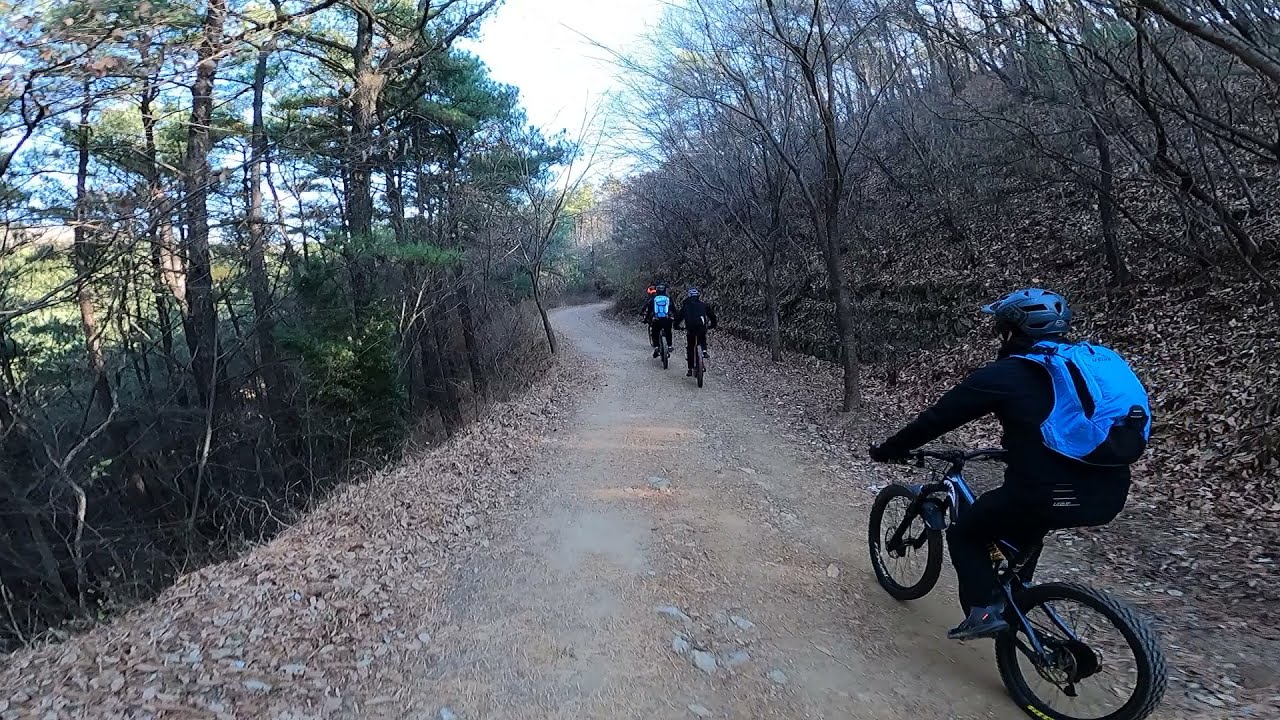Three mountain bicyclists are seen ascending an upward-sloping dirt trail through a dense forest with compacted light brown soil. The path is dotted with white rocks and bordered by dead leaves and branches, which intensify the rustic, natural setting. The scene appears to be sunlit, with rays filtering through the trees that form a natural wall along either side of the trail. The rider closest to the camera is on a blue bike with black wheels and is dressed entirely in black, accentuated by a blue backpack and a blue helmet. In front of this person, another cyclist dons a black jacket, black pants, and a gray helmet. Leading the group, the third cyclist, similarly attired in black, also carries a blue backpack. The image, taken from behind the cyclists, captures the essence of a challenging and steeply inclined forest trail.